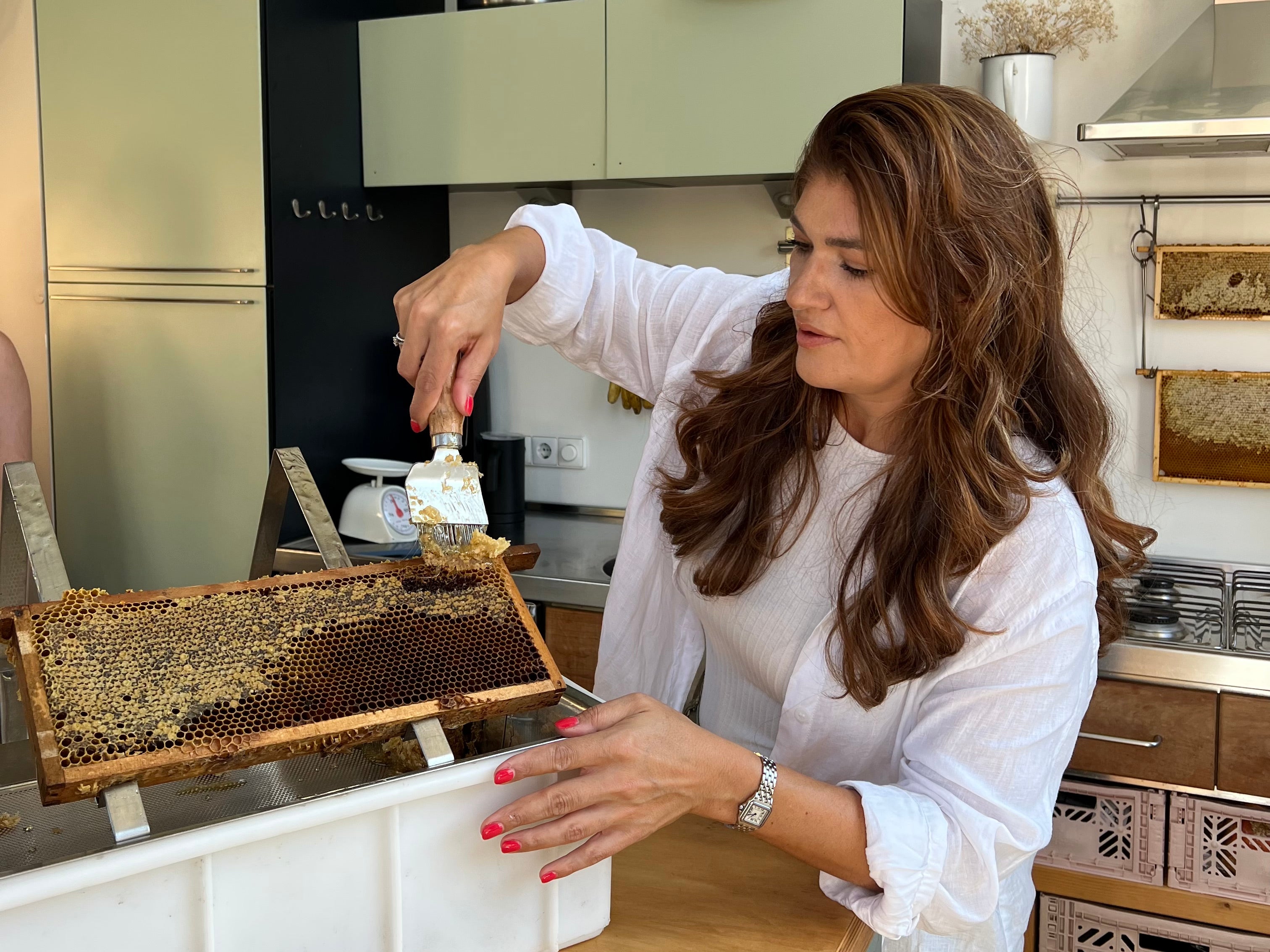This detailed photo captures a middle-aged Caucasian woman with long, wavy, light brown hair standing in her modern kitchen, which features a wood and mint color scheme and green cabinets. She wears a white button-up dress shirt that is undone, revealing a white tank top underneath. Her nails are painted a peachy pink, and she sports a silver watch and a wedding ring on her left hand. Positioned at the far end of a circular wooden table, she holds a plastic tote in her left hand. Inside the tote, partially protruding, is a rectangular section of a beehive with a honeycomb, dripping a honey-colored substance. She uses a specialized scraper tool with pointy, comb-like ends to extract the honey. Behind her, additional beekeeping screens that appear to have honey already scraped off hang above her stove, contributing to the beekeeping activity shown in the image.